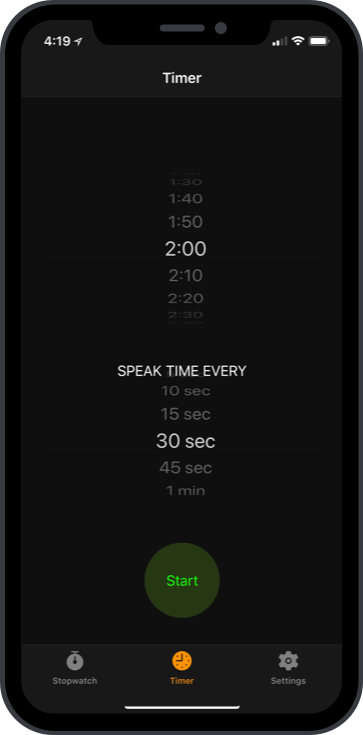This detailed caption describes the image's content concisely and effectively focuses on the key visual elements and their arrangement on the smartphone mock-up screen:

---

The image showcases a detailed mock-up of a recording app interface on a smartphone, closely resembling an iPhone. At the top of the screen, the status bar displays the time "4:19" on the left, two out of four signal bars, full Wi-Fi connectivity, and a fully charged battery icon. Below this, the timer interface features a faux 3D spinning clock with time markers at 10-minute intervals: "1:30", "1:40", "1:50", rendered in light gray, and "2:00" in white, followed by "2:10", "2:20", and "2:30" depicted as curving away. 

Adjacent to the clock, there are selectable speech time intervals listed as "10 seconds", "15 seconds", "30 seconds", "45 seconds", and "1 minute". The "30 seconds" interval is highlighted, indicating it is currently selected. A prominent round, green button with a brighter green center labeled "Start" is displayed below the timer options.

At the bottom of the screen, navigation options include "Stopwatch" and "Timer", with a gear icon for settings. The screen is contained within the phone's bezel, which is black on the outer edge transitioning to a silver metallic or plastic frame, typical of an iPhone design.

The mock-up rests on a white background, emphasizing the screen's interface and the smartphone's design details.